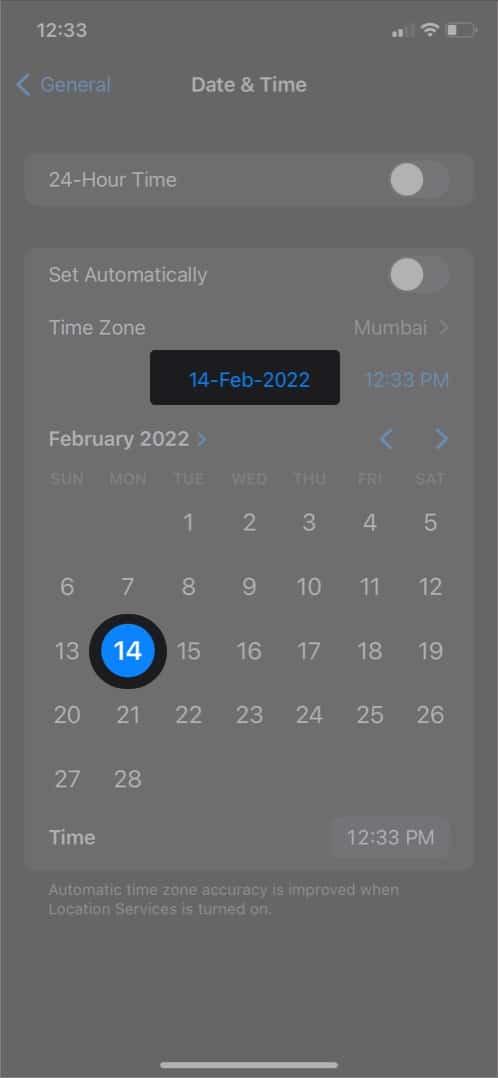This screenshot from a cell phone displays the 'Date & Time' settings screen against a dark gray background. At the top of the screen, the status bar shows it is 12:33 p.m., the user has two bars of cellular coverage, active Wi-Fi, and a very low battery. Below the status bar, a blue back arrow points to the left next to the word "General." 

Under "Date and Time," the settings panel is presented including the 24-hour time option, which has the slider switched off. The "Set Automatically" option also has its slider turned off. The time zone is set to "Mumbai," and the date displayed is "14 February 2022." This information is rendered in blue text within a black rectangle.

A horizontal layout of the days of the week is visible, starting with Sunday and ending with Saturday. The month of February 2022 is shown, with each day of the month appropriately positioned. Notably, February 14th is highlighted with a thick blue circle enclosing the date number, "14," which is displayed in white.

Below the calendar, the current time is reiterated as "12:33 p.m." and a note explains that "Automatic time zone accuracy is improved when location services are turned on."

The image has no people and is wider than it is tall, providing a thorough view of the settings page.